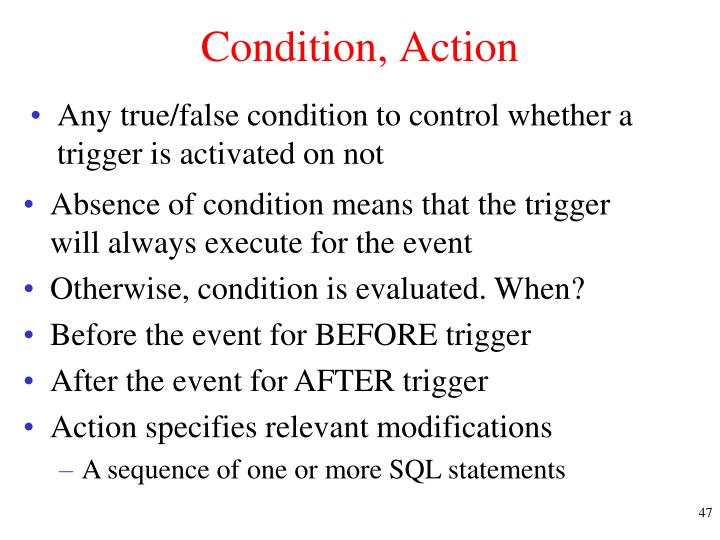The image depicts a PowerPoint slide with a plain white background. Centered at the top in red text, it reads "Condition, Action." Below this heading, there are six bullet points, each marked with a small blue bullet on the left side, and the text is written in black, serif font, likely Times New Roman. The bullets convey the following information:

1. Any true/false condition to control whether a trigger is activated or not.
2. Absence of condition means that the trigger will always execute for the event.
3. Otherwise, condition is evaluated when.
4. Before the event, for BEFORE trigger.
5. After the event, for AFTER trigger.
6. Action specifies relevant modifications.

   - A sequence of one or more SQL statements.

In the bottom right corner of the slide, there is a small number "47."